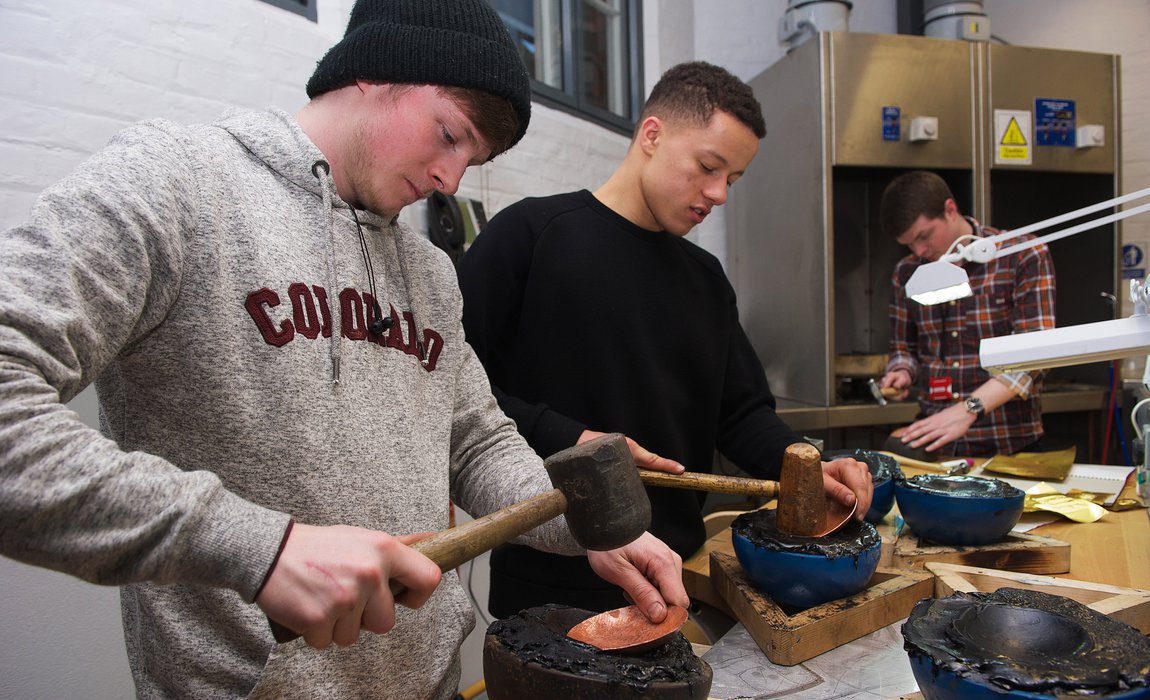The image showcases three young men, likely teenagers, engaged in a metalworking project possibly in a school workshop. The young man on the left, wearing a gray hoodie with 'Colorado' printed in dark reddish-brown letters, is intensely focused on hammering a copper or bronze disc. He wields a wooden mallet in his right hand. In the center, a young man in a black sweater also hammers a similar metal disc, working to create a curved shape in a bowl-like mold. The third young man in the background, dressed in a plaid button-up shirt, participates in the same activity, positioned near a large cabinet, a window, and a white concrete brick wall. The scene indicates a structured learning environment, with all three boys concentrating on shaping the metal under guided instruction.